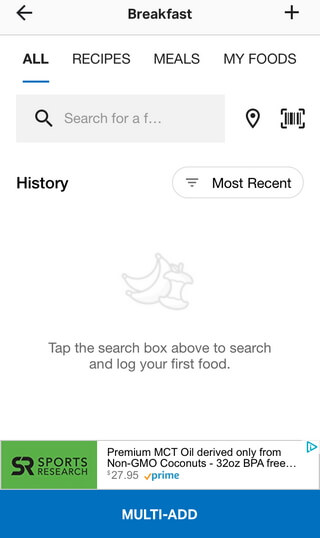The image depicts an app interface for logging food intake, specifically focused on breakfast. The top of the screen features a gray bar. On the far left of this bar is a backward arrow, presumably for navigating to a previous page or meal selection. Centered in bold text is the word "Breakfast," and on the far right is a plus sign, likely for adding a meal.

Below the gray bar is a menu with options written in all capital letters: "ALL" (underlined), "RECIPES," "MEALS," and "MY FOODS." Directly beneath this menu is another gray bar containing a magnifying glass icon, which suggests a search function for finding specific foods. Next to the search bar are symbols: a landmark icon, possibly for indicating the location where the meal is consumed, and a barcode icon for scanning packaged foods.

Following this, there is a section with two bolded but non-caps text options: "History" and "Most Recent," the latter accompanied by an upside-down triangle, the function of which is not specified. The main body of the interface is a large white area with a faded, stylized image depicting bananas and an apple core. Overlaying this image is a grayed-out text prompt: "Tap the search box above to search and log your first food."

At the bottom of the screen, there is an advertisement for Sports Research. The ad's logo, located at the top left, is in green with the letters "SR" interconnected. The ad text is black on a white background and promotes "Premium MCT Oil derived only from non-GMO coconuts" in a 32-ounce BPA-free container, priced at $27.95. An Amazon Prime logo with a blue check mark and a blue triangle appears next to the price. The ad's bottom section is a blue banner with white, all-capital text, reading "MULTI-AD."